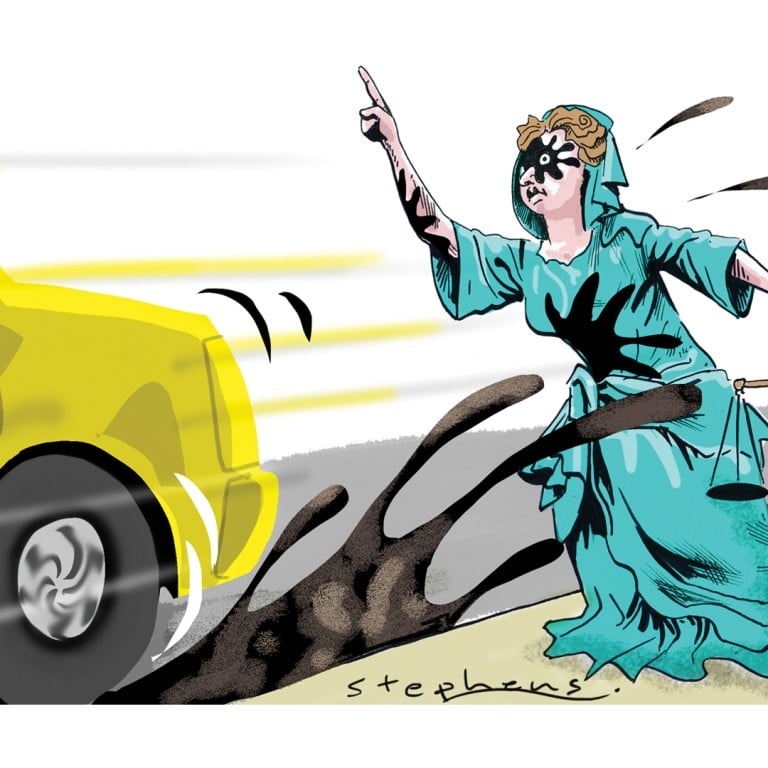The image is a detailed cartoon drawing of a woman in a turquoise or green, hooded dress, striking a resemblance to the Statue of Liberty. Her finger is raised, possibly suggesting she's trying to hail a taxi. Her dress is long and robe-like, giving it a wizard or witch-like appearance. She stands on a mound of dark beige grass, near a road that transitions from a gray asphalt surface to brown dirt beneath. A yellow car is depicted speeding past her, its motion indicated by action marks and yellow trails. One of its tires is visible while it kicks up a splash of black mud, oil, or gasoline, which covers the woman's face and body, leaving her noticeably upset. The illustration is signed at the bottom with the name "Stevens," underlined.